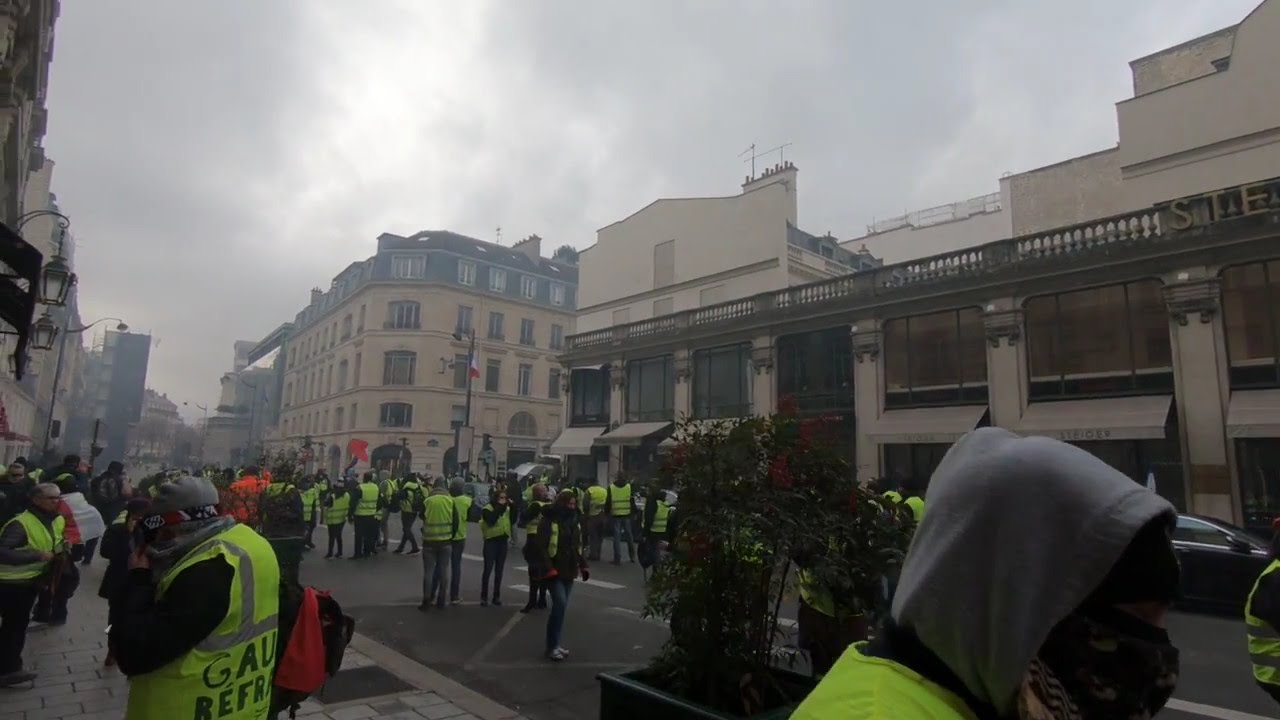The photograph captures a bustling Parisian street in what appears to be a European city, featuring classic old Continental European style buildings made of cement, mortar, and brick, standing between two and four stories high. The street is mostly devoid of car traffic, with just a few cars parked along the sides, but is crowded with people wearing bright yellow reflective vests. These vests have some writing on the back, although the exact lettering is partly obscured. 

The scene suggests these individuals might be part of a demonstration or event, as they are spread out both in the street and on the sidewalks, seemingly managing the crowd or preparing for some activity. The photograph is taken from an angle that showcases the middle of the street, emphasizing the crowd and leading the eye towards the buildings in the background, which feature historic railings and curved corners, adding to the old European charm.

Visible in the bottom right corner of the photo is a person dressed in a gray hoodie with part of their reflective vest showing. The people in the image are dressed in basic pants and sweatshirts, suggesting a chilly day. Additionally, a planter with red flowers adds a splash of color in the otherwise muted urban scene. Overall, the image feels vibrant and alive, capturing the essence of an active street in a historical city.